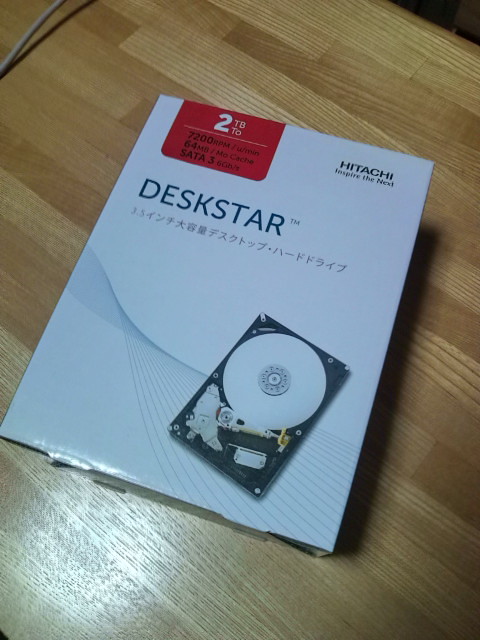The image showcases a retail box for a Hitachi Deskstar hard drive prominently placed on a medium to light brown wooden surface. The box features an image of the hard drive, where you can see the internal components, including the platter and the hardware. The packaging highlights key specifications such as 2 terabytes of storage, 7200 RPM speed, 64 MB cache, and SATA 3 interface. The brand name "Deskstar" is in large, black capital letters, and below it, there are Japanese characters. The box also includes the phrases "Hitachi" and "Inspire the Next." The package is predominantly white with a red label at the top and contains wavy blue lines in the background.